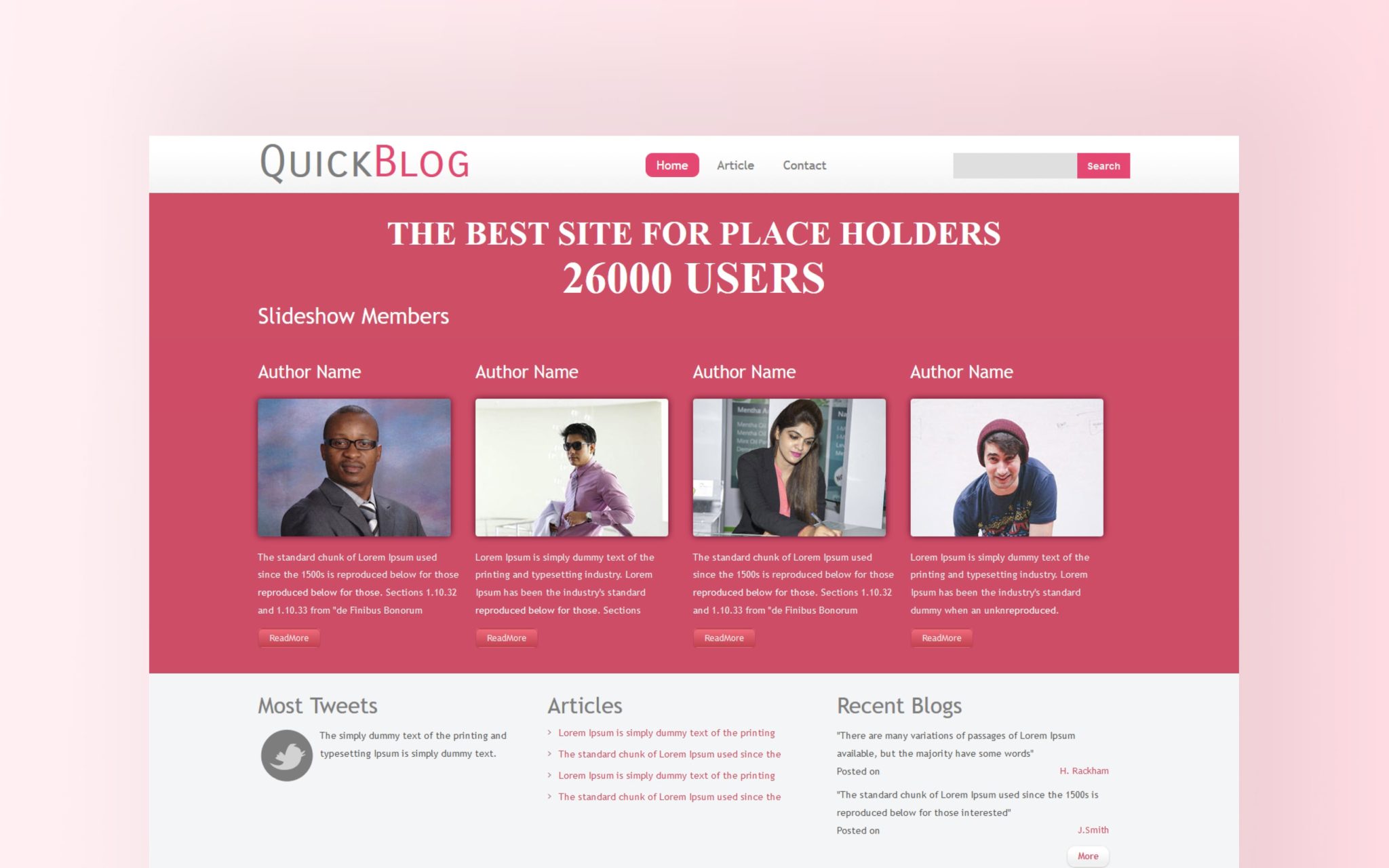The screenshot features a webpage with a light pink background. At the bottom center, there's a large white square. At the top left of the page, the logo "Quick Blog" is displayed, with "Quick" in gray and "Blog" in red. To the right, there is a navigation bar that includes a red 'Home' button with white text, followed by white 'Article' and 'Contact' buttons with gray text, and a pink search bar.

Beneath the navigation bar, a rosy salmon-colored rectangle is prominently featured with white, centered, all-caps text that reads "THE BEST SITE FOR POLICYHOLDERS." Directly below that, in slightly larger white text, it states "26,000 USERS."

Further down, there’s a section titled "Slideshow Members" in white text, followed by another line two rows down with "Author Name" repeated four times, each aligned with a picture of the respective author below. Each picture is followed by a brief description in white text, and to the left of these pictures, there are pink buttons with white text.

Below this section, the background transitions to light gray, comprising three columns with headers in gray text: "Most Tweets" on the left, "Articles" in the middle, and "Recent Blogs" on the right.